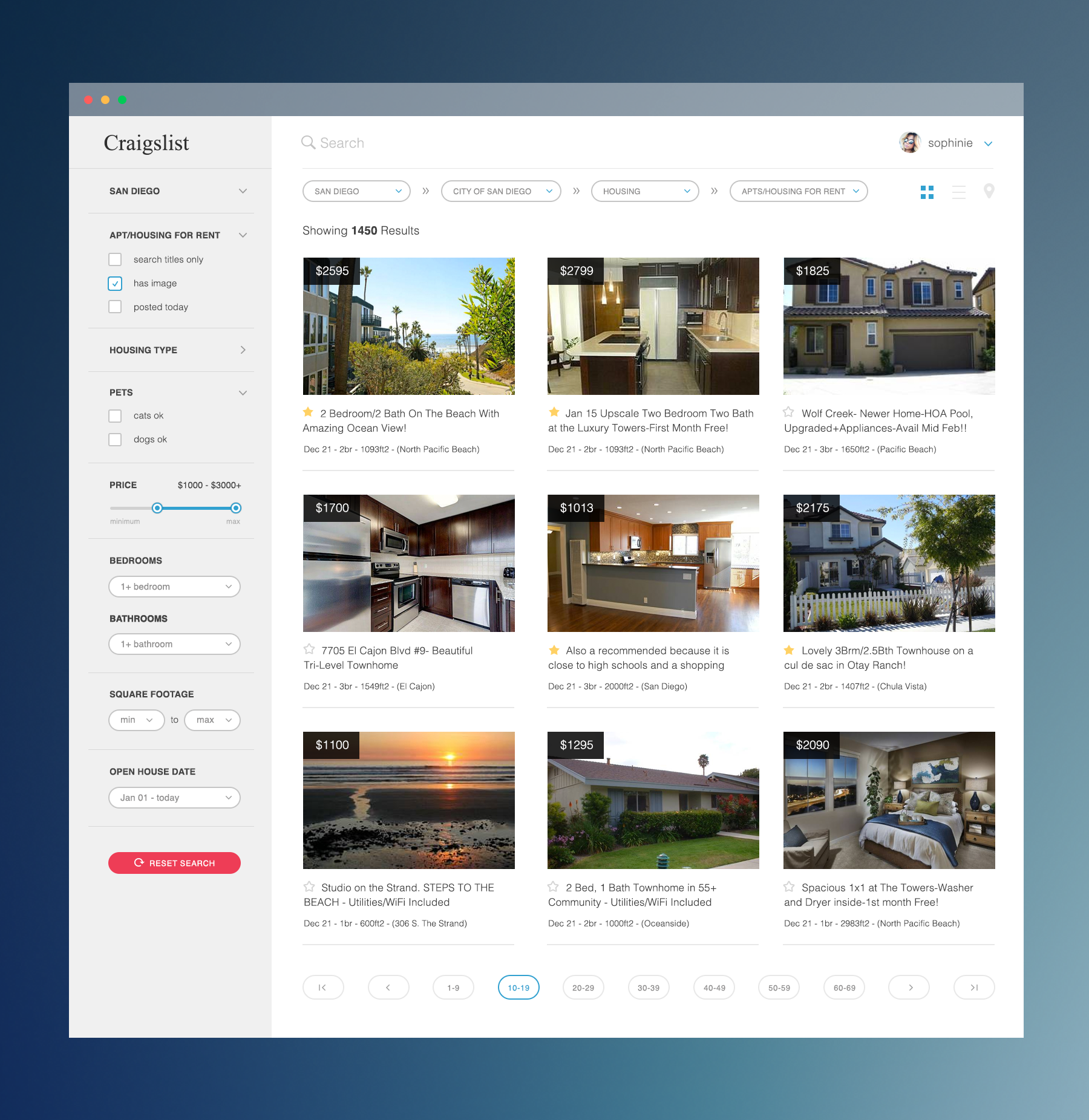The image is a large, square photograph with a gradient blue background that transitions from dark blue on the left to light blue towards the lower right corner. At the center of the image is a screenshot of a Craigslist page. The top of the screenshot features a dark grey banner bar with three circular dots on the left side: red, yellow, and green.

Directly below the banner, the Craigslist page is visible. On the left side of the page, there is a vertical grey panel extending to the bottom. At the top of this panel, the word "Craigslist" is displayed in black font, followed by the word "San Diego" with a city drop-down box next to it for changing locations. 

Beneath the city selector, the panel contains various filtering options, including "housing for rent" with three check boxes, followed by "price range," "posted today," and "housing type," which has an unexpanded arrow next to it. Further down, there are options for filtering by "pets," "price" with an adjustable slider bar, "bedrooms," "bathrooms," "square footage," and "open hours." At the bottom of the panel, there is a red "reset search" button.

To the right of the grey panel, the main section of the page displays nine property thumbnails arranged in a grid. Below each thumbnail, there are descriptions of the respective properties. At the bottom of this section, there are navigation controls, including ovals with forward and backward buttons and page number indicators. The page numbers are grouped in ovals, ranging from 1-9, 10-19, and so on.